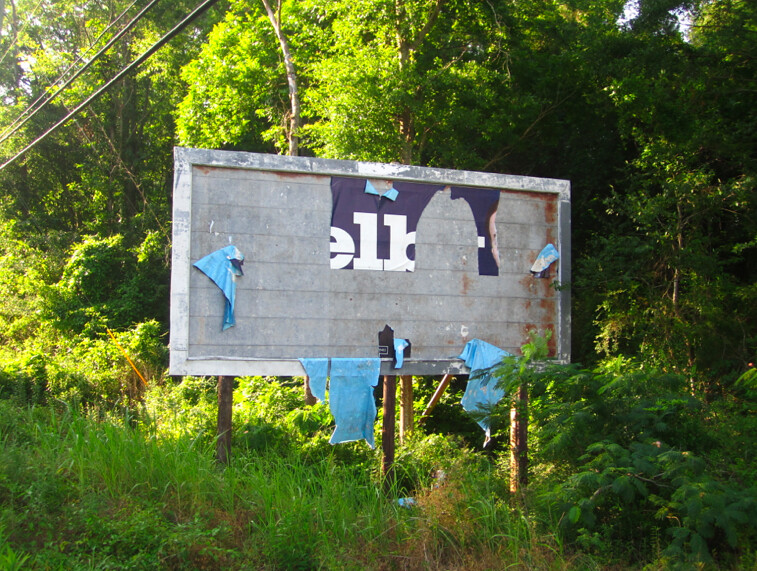The photograph features a dilapidated billboard situated in a seemingly untouched wilderness area, surrounded by an abundance of nature. Towering deciduous trees dominate the landscape, with the odd evergreen and an undergrowth of tall, unkempt grass. In the lower right foreground, a couple of vibrant green bushes add a splash of color to the otherwise wild setting.

The billboard itself is mounted on a structure of wooden posts—three visible in the front, with additional supports likely hidden at the back. The billboard, a horizontally oriented rectangle, once sported a white painted border, now largely peeling and weather-worn. The majority of the billboard's original content has eroded, leaving behind a gray, textured surface that vaguely resembles concrete blocks, though it is likely made of a lighter material. 

Brown stains streak down the right-hand side of the billboard, adding to its forlorn appearance. Torn remnants of paper or vinyl cling to the billboard, with three significant strips draping down and fluttering in the breeze. One of the remaining pieces bears the letters "ELB" in white against a blue background, hinting at its past message. The scene is one of decay and neglect, isolated in a tranquil wilderness.